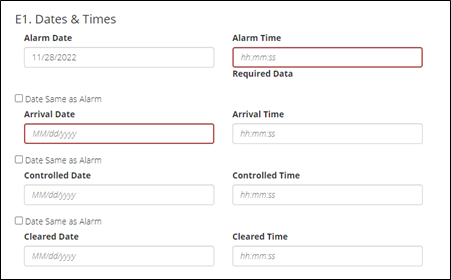Screenshot of the "E1.Dates and Times" Interface:

The image displays a section of a software interface called "E1.Dates and Times," featuring a black, one-pixel thin border surrounding the entire area. At the top, on the left, is the "Alarm Date" field with a placeholder text showing a date in the format "MM-DD-YYYY" (e.g., 11-20-2020 or 2022), encased within a light gray outline. To the right of this is the "Alarm Time" field designated for hours, minutes, and seconds, labeled "HHMMSS" with placeholder text "HH:MM:SS." This field is highlighted in a brownish or reddish color, indicating it is required data.

Below these, on the left side, is an unchecked checkbox labeled "Date Same as Alarm." Adjacent to it is the "Arrival Date" field, which follows the "MMDDYYYY" format. To the right of this checkbox is the "Arrival Time" field in the "HHMMSS" format. The "Arrival Date" field on the left is also highlighted in brown, while the other input fields on the screen are in gray.

Beneath these, on the left side, is another unchecked checkbox labeled "Date Same as Alarm." Below it is an unchecked checkbox labeled "Same as Below," also succeeded by another checkbox labeled "Date Same as Alarm." Next to these, the left column lists "Control Date" and "Clear Date" fields, both using the "MMDDYYYY" format. To the right, the corresponding "Control Time" and "Clear Time" fields are in the "HHMMSS" format. All eight input fields feature bold black text, ensuring clear readability.